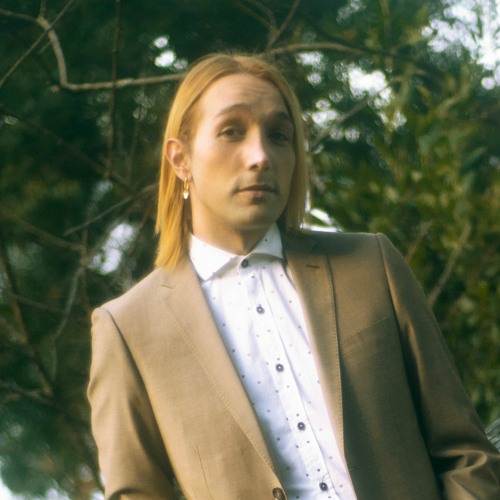In this portrait, a young Caucasian man with vibrant, shoulder-length blonde hair, parted down the middle, looks directly at the camera with raised eyebrows and a neutral expression. He is dressed in a stylish ensemble consisting of an open, light brown blazer over a white button-down shirt adorned with black polka dots. His slim frame occupies much of the image. Accessories include a hoop earring with a diamond-like jewel in his right ear. The background features a softly focused, blurred scenery of green foliage, tree branches, and patches of blue sky that add a natural element to the soft, vintage feel of the photograph.